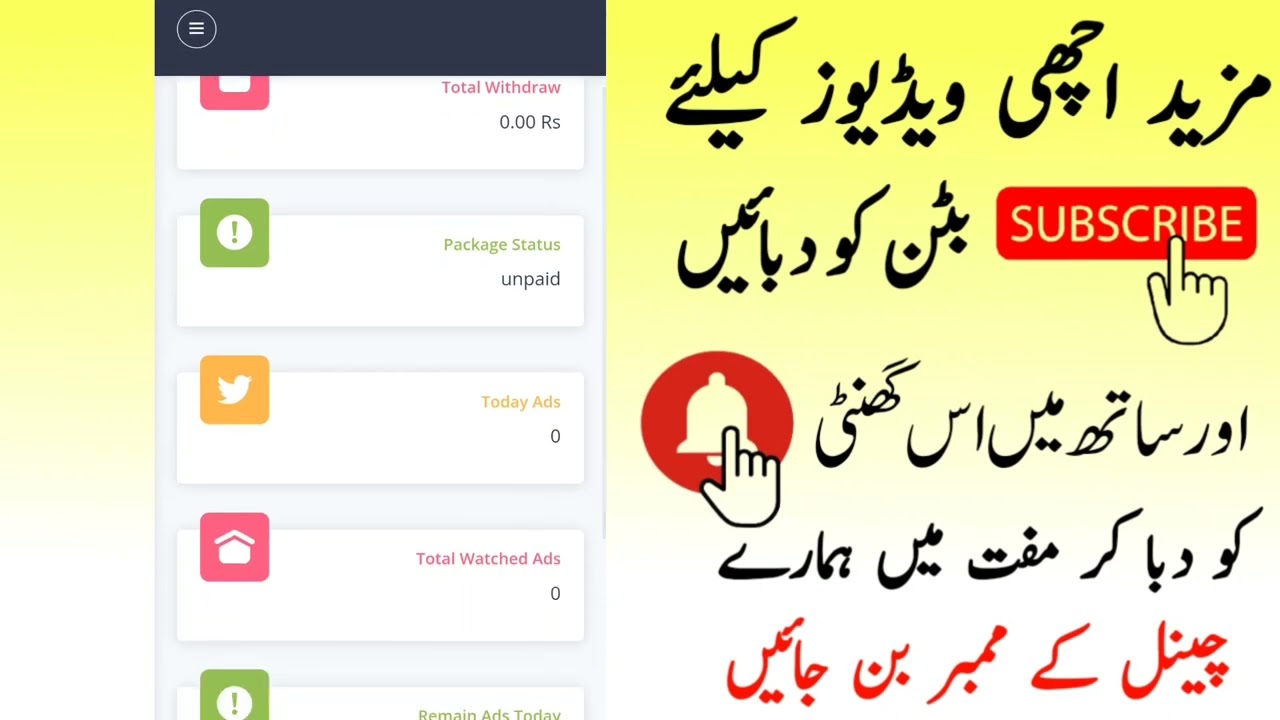The image features a pale yellow background that gradually transitions to a darker yellow towards the top. In the upper right corner, there is a prominent red "subscribe" button with a hand icon pointing towards it. Centrally located is a red circle with a white bell, also accompanied by a hand icon. The image contains various texts in different languages and styles: large black script at the top, slightly smaller black text in the middle, and red text at the bottom. On the left side, there is a rectangular inset resembling a mobile device screenshot, featuring a black bar on top and a gray background. This inset showcases multiple interactive options such as "total withdraw," "package status," "today ads," "total watched ads," and "remain ads today," each with corresponding icons in pink, green, and orange. This composition serves as a YouTube video thumbnail, capturing attention with its colorful and detailed elements.